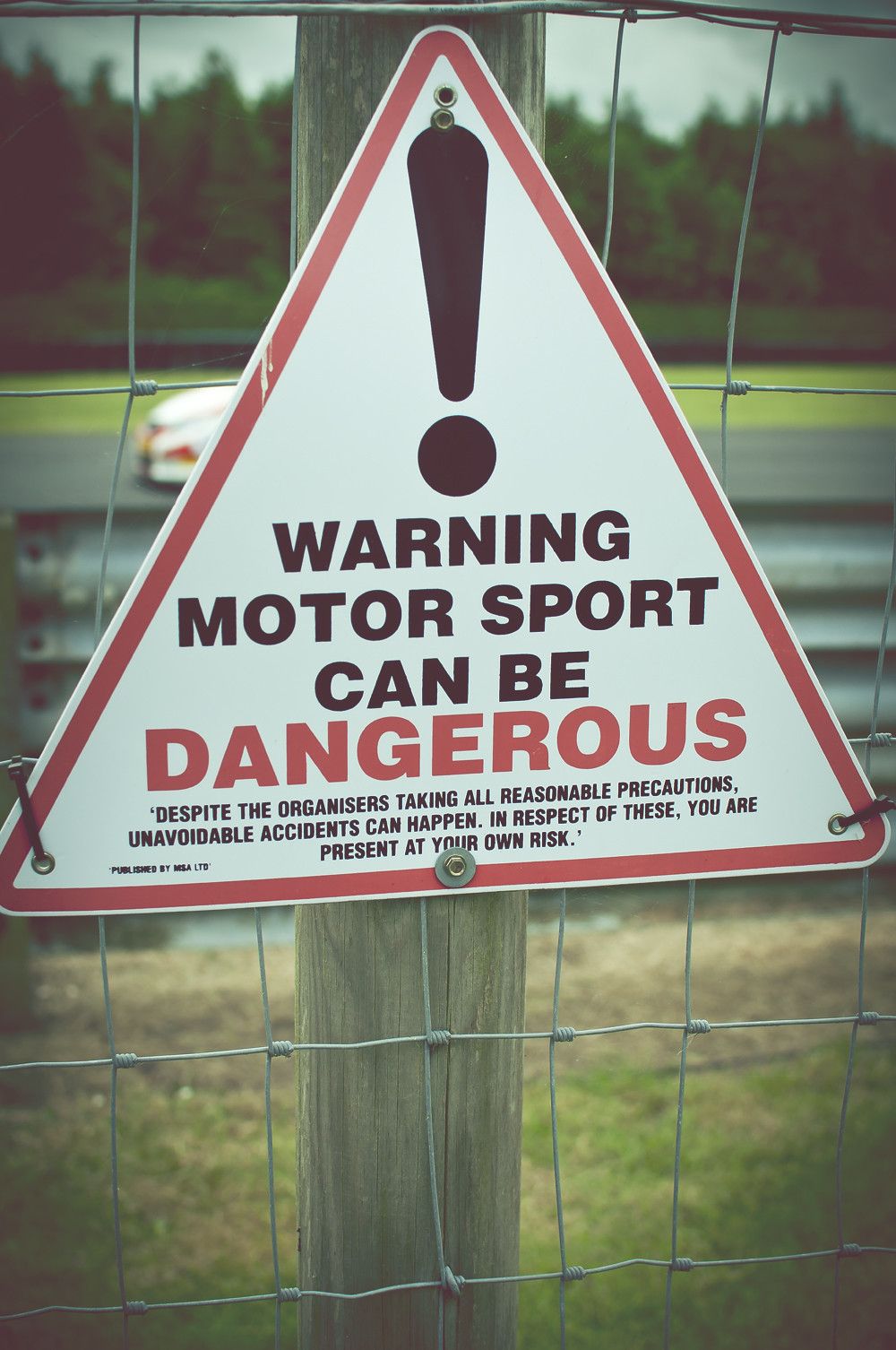The image showcases a detailed view at a racetrack setting, prominently featuring a triangular warning sign. The sign, nailed to a brown wooden post and secured with black zip ties, stands in front of a rugged silver gate-like fence, characterized by mesh wire. The sign itself is white, bordered by a striking red outline with a large black exclamation point at its apex. Below the exclamation point, in bold capital letters, the sign reads: "WARNING, MOTORSPORT CAN BE DANGEROUS," with the word "DANGEROUS" highlighted in red. The cautionary message continues in smaller black letters: "DESPITE THE ORGANIZERS TAKING ALL REASONABLE PRECAUTIONS, UNAVOIDABLE ACCIDENTS CAN HAPPEN. IN RESPECT OF THESE, YOU ARE PRESENT AT YOUR OWN RISK."

Behind the fence, a racetrack unfolds, featuring a white car on a dark gray track, flanked by a silver guardrail. Encompassing the setting are patches of green and yellow grass, along with dense clusters of trees and bushes under a partially overcast, slightly blue sky. This vivid backdrop emphasizes the precarious nature of the motorsport event occurring, underscoring the critical warning presented in the foreground.